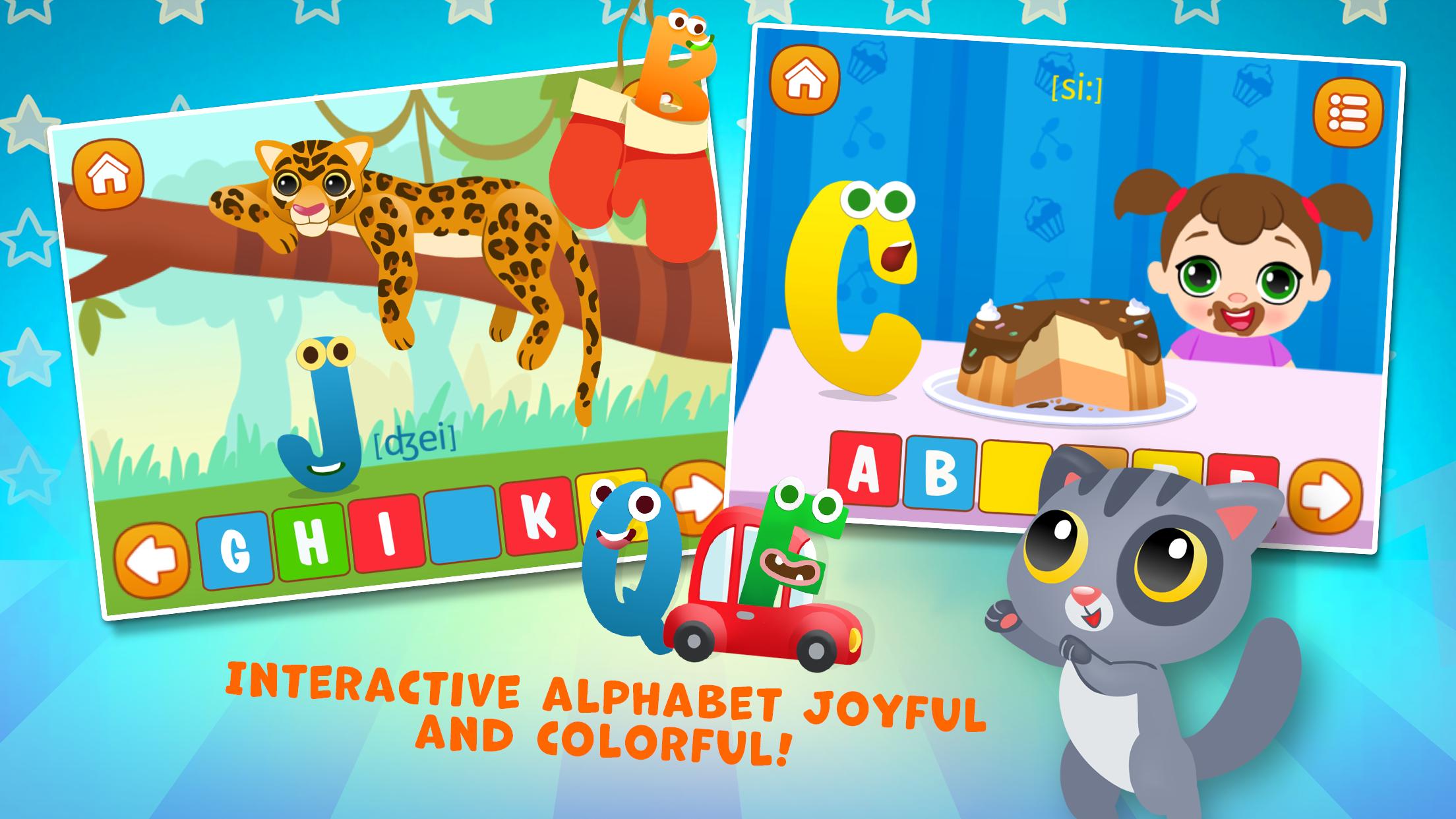The image features a vibrant blue background adorned with the bottom halves of stars, some gray and some blue, scattered along the top and left edges. Within this backdrop are two distinct, detailed illustrations. 

The first illustration showcases a playful collage. A leopard leisurely lounges on a large tree limb. Nearby, a small box depicts a house situated in the left corner. Below it, two red gloves are illustrated beside a whimsical bee with animal-like eyes. A blue letter 'J' with eyes adds a quirky touch. Additionally, a brown box with a white arrow pointing left is included, along with the letters G, H, I, and K, each in a different color.

The second illustration is equally detailed. It features a large, yellow letter 'C' with expressive eyes and a nose. Beside it, a plate holds a cake, and a little girl with pigtails and chocolate smeared around her mouth stands nearby. Above her, a square at the top of a house is visible along with another square marked by three lines and dots. Colorful letters A, B, and C are displayed along the bottom. The illustration also includes a small red car driven by a green character, a blue letter 'Q' with eyes, and a small gray cat. The image is interspersed with the words "interactive," "alphabet," "joyful," and "colorful," enhancing its playful and educational nature.